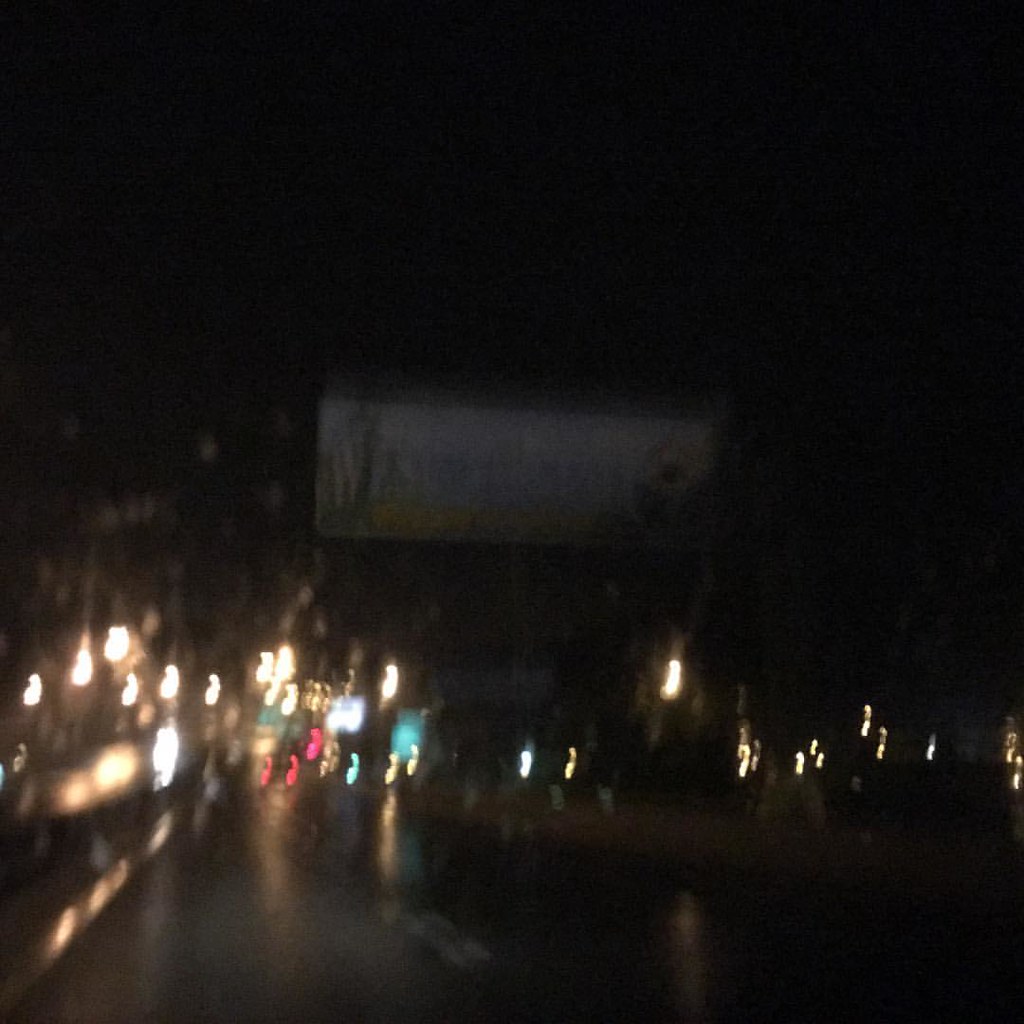The photo depicts a very blurry nighttime scene. The sky overhead is completely dark, devoid of stars or any discernible celestial features. The focal point in the center appears to be a large, indistinct billboard or banner, though the text or image it carries is unclear due to the blurriness. At the bottom of the image, a smattering of blurry lights in white, pink, and teal blue suggests the presence of a road or street, which appears to be wet, hinting at recent rain. These lights might also include some hanging from trees, contributing to the ambient glow. The overall image is not very sharp, making it difficult to pick out precise details, but the general impression is that of a misty, damp night scene with various colorful lights adding to the subdued atmosphere.